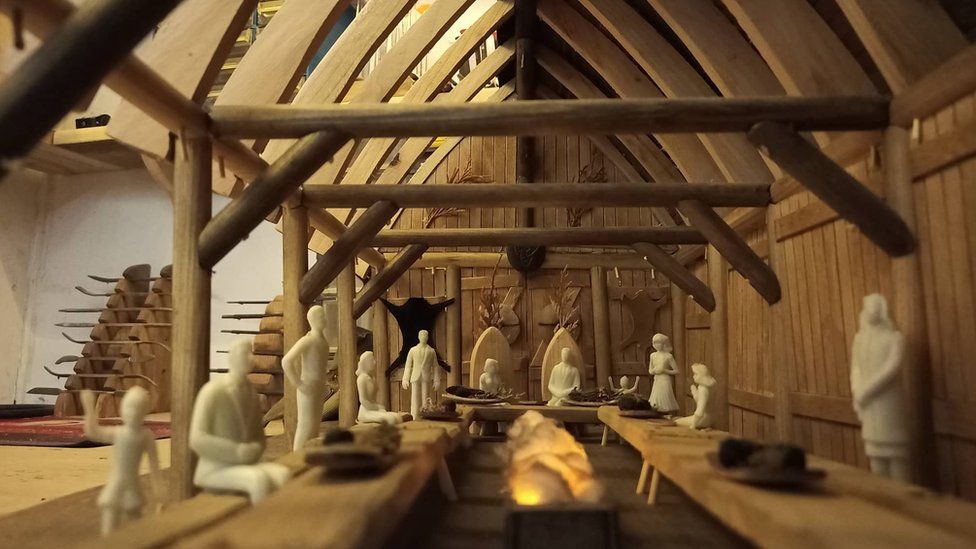This image depicts an intricate art display inside a museum, meticulously crafted to resemble the interior of an ancient castle or a barn-like structure with a refined aesthetic. The scene is set within a wooden building characterized by a triangular, angular roof and a mix of dark and light wood elements. Dominating the center is a long, rectangular table surrounded by carved figures, possibly made from wood or resin, engaged in what appears to be a ritual or communal gathering.

On the left and right sides of the table, long, rectangular benches form a horseshoe shape, with various figures either standing or seated. In the middle of the table, there is a striking rectangular fire made from a cottony material illuminated by lights, giving it a glowing, golden appearance. Arranged around the table, these statues create a lifelike scene; one statue to the left appears to be waving.

Against the wooden wall on the right, a white sculpture of a person stands with crossed arms. Toward the background, a head table features statues of a man and a woman seated on large, throne-like chairs, possibly representing royalty. Directly beside them, other figures are positioned: three children stand at the table's end, while a man stands against the wall behind a bearskin rug, next to the queen's chair. 

Further to the left, a woman is seated, adding to the tableau's complexity. This detailed scene captures the essence of a historical or ceremonial gathering, inviting viewers to immerse themselves in the elaborate craftsmanship and storytelling of the display.